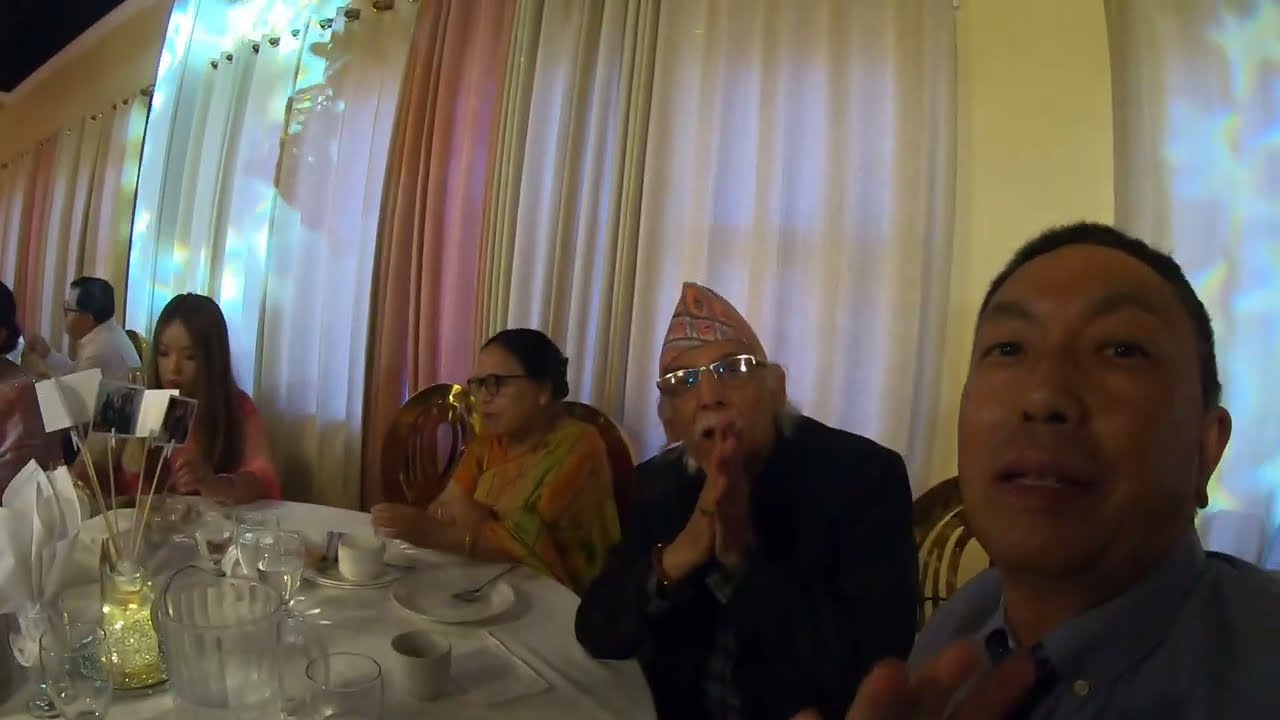In a lively and colorful restaurant setting, a group of Asian people are gathered around a table adorned with a white tablecloth and elegant tableware. The centerpiece consists of a jar filled with fairy lights and photographs held by clips, adding a personal touch to the atmosphere. On the far right corner of the table sits a man in his 30s to 40s, next to an older man wearing glasses and a scarf on his head. Beside the older man is a woman of similar age with dark hair pulled into a bun, wearing dark glasses and a vibrant, colorful top. Around the curve of the table sits a younger woman, with brown hair and a bright pink shirt, her age difficult to determine but she could be anywhere from 12 to 30. Behind the group, drapes in shades of pink, yellow, and creamy white add a soft backdrop, possibly reflecting light that resembles water. The scene suggests a formal celebration or gathering, with everyone dressed in their finest and directed attentively towards the camera, creating an intimate and memorable moment.